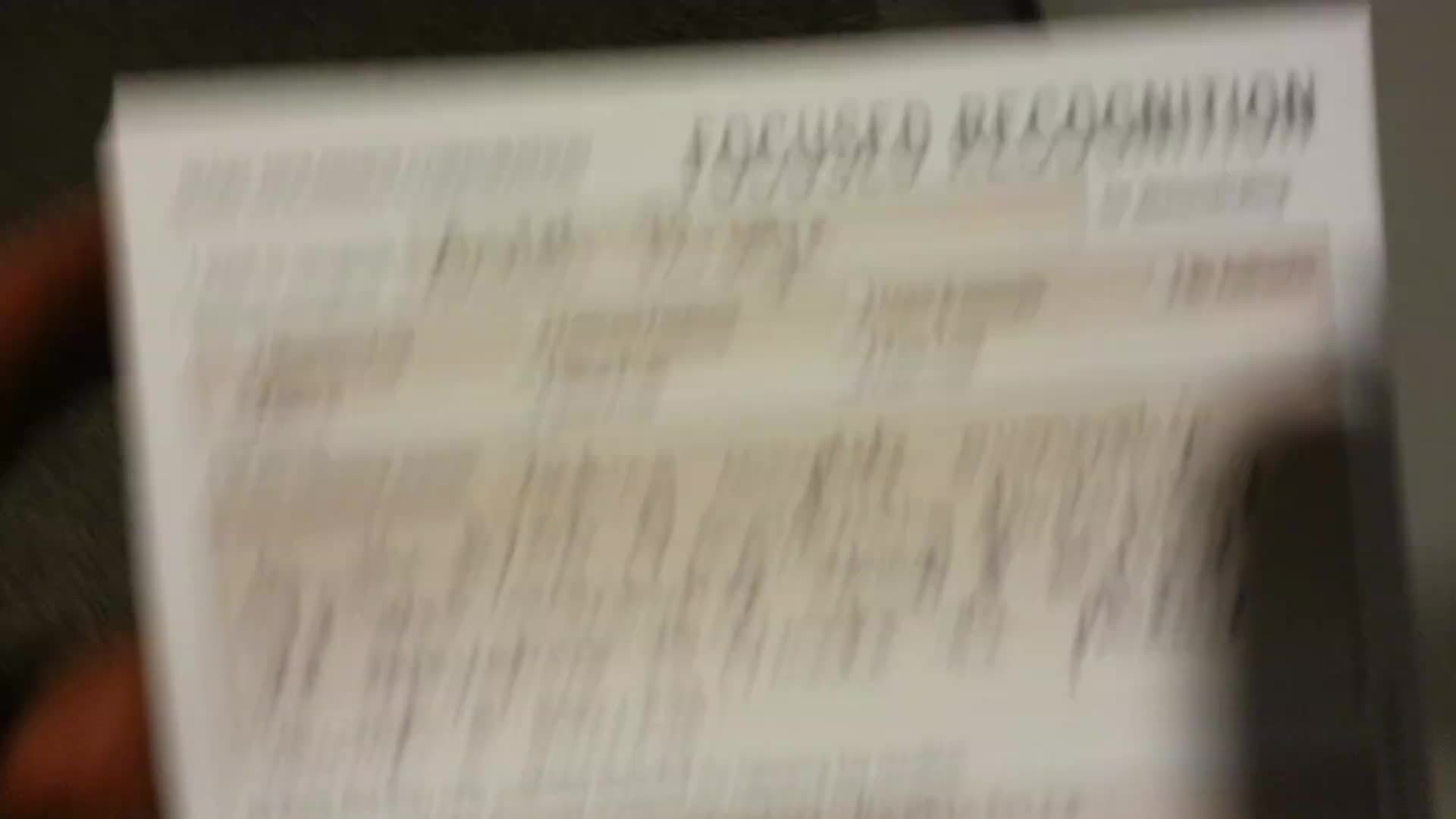This is a horizontal, rectangular color photograph that is very blurred. Central to the image is a white paper slip, which is held by two fingers visible on the left side of the photograph. The majority of the background is black, with a noticeable black strip or shadow in the lower right-hand area. The paper appears to feature various sections of text; in the upper right corner, the words "Focused Recognition" are legible. Below and to the left of this legible text, there is what appears to be multiple lines of cursive writing and possibly a paragraph, although the exact details are indiscernible due to the blurriness. The text on the paper is black, and despite the clarity of individual characters, the overall content remains unreadable. In the upper left corner of the paper, there is a portion of typed text.